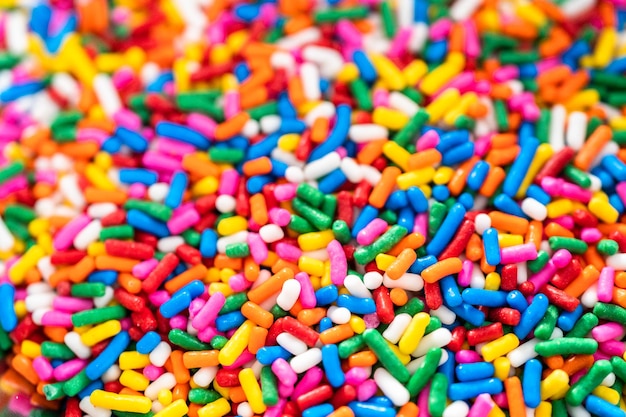This is a close-up, horizontal photograph of an assortment of colorful candy sprinkles. The image, nearly twice as wide as it is tall, showcases a vibrant mix of small cylindrical pieces of candy, resembling those used on cakes, ice cream, and cupcakes. The candy sprinkles come in a variety of colors, including yellow, light blue, green, orange, red, white, and pink. These sprinkles, rounded at the ends and differing slightly in size, are in sharp focus primarily in the center and right side of the image, with a noticeable blur towards the upper left corner and across the top due to a shallow depth of field. The overall effect is a dynamic sea of colorful, candy-coated sprinkles spreading across the frame.